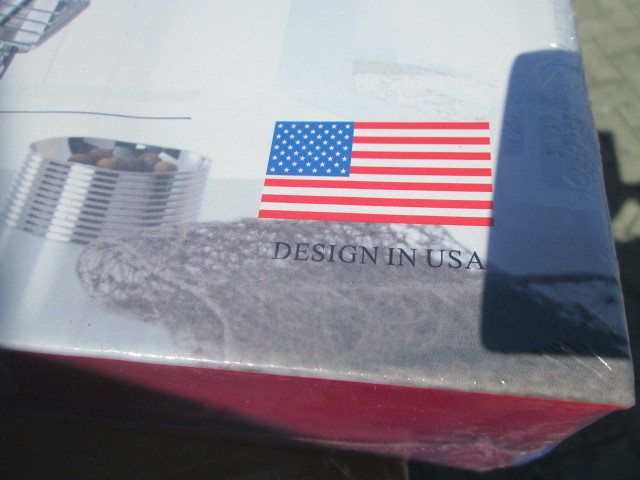The image depicts a box of an unknown product, photographed outdoors on a surface that includes brick pavers and a patch of green ground in the top right corner. Predominantly light grey, the box features a maroon side closest to the viewer and a visible shadow cast by the cell phone used to take the photo on the right-hand side. In the center of the box is an American flag with the text "DESIGN IN USA" below it. To the left of the flag, there is a stack of metallic round discs, with the top one appearing to contain chestnut-like objects. Below the flag, there is a brown mesh detail resembling a hunting blind drape. Additionally, a blue stripe is visible on the right side of the box.